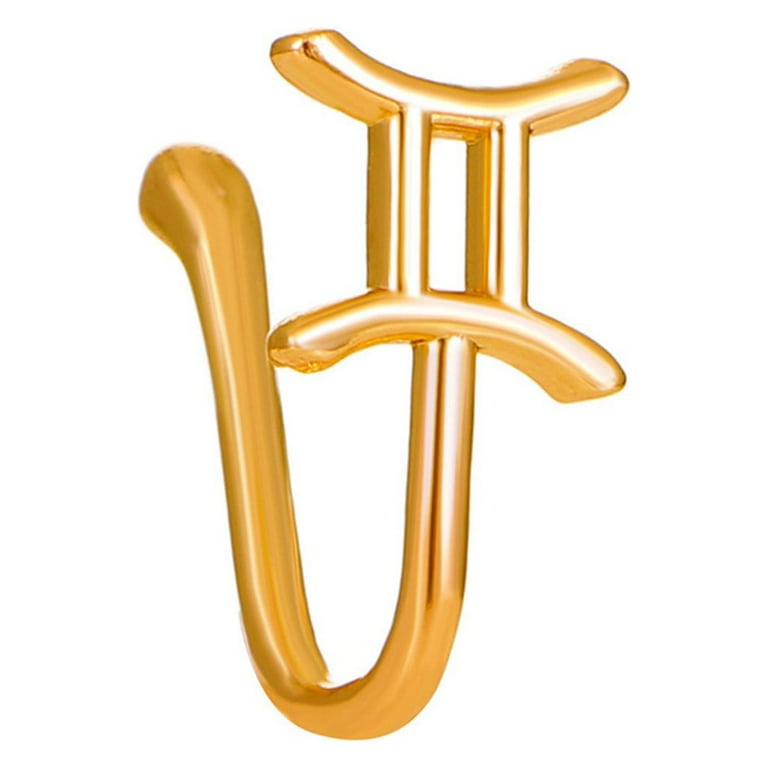Against an all-white background, the image showcases a gold-colored hook designed for hanging items like coats. The hook is shaped in a U or J form with highly reflective gold material. At its mounting end, the hook features a bulbous, knob-like tip. Further up, the hook displays a unique design element: a Roman numeral "Ⅱ" prominently featured at the top, with each end of the numeral curving slightly upward and downward, respectively. The central part of the hook forms an open rectangle with extensions on either side. The entire design, with its intricate detailing and reflective surface, creates a visually striking yet elegant gold hook.